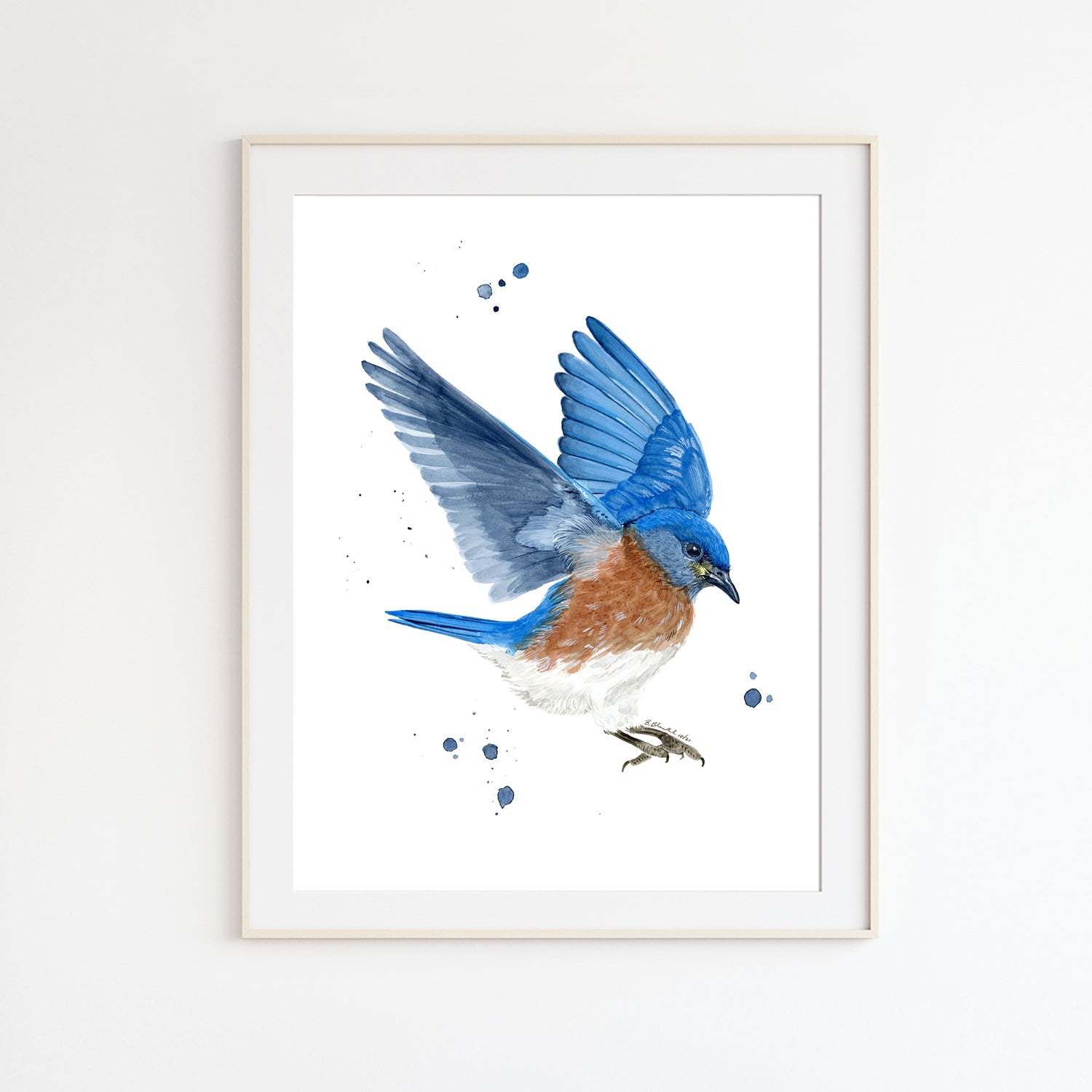The piece is a watercolor painting of a bluebird captured in mid-landing, meticulously framed in a white wooden frame against a plain white wall. The bird is primarily blue, featuring striking blue wings that are extended downwards as it prepares to alight. Its head is also blue, with focused eyes, while its underbelly transitions from a brown neck and chest to a white lower belly. The bird's claws, appearing dark brown or black, are splayed open, ready to grasp something beneath it. The background within the frame is stark white, accentuating the bird's vibrant colors. Surrounding the bluebird are various splotches of blue paint, with a large splotch directly to the right, three below the tail, two above the wings, and several smaller blue and black dots dispersed around these larger ones. The absence of any other elements in the painting leaves the location of the bird ambiguous, allowing viewers to imagine it free in the open air or potentially confined in an aviary.